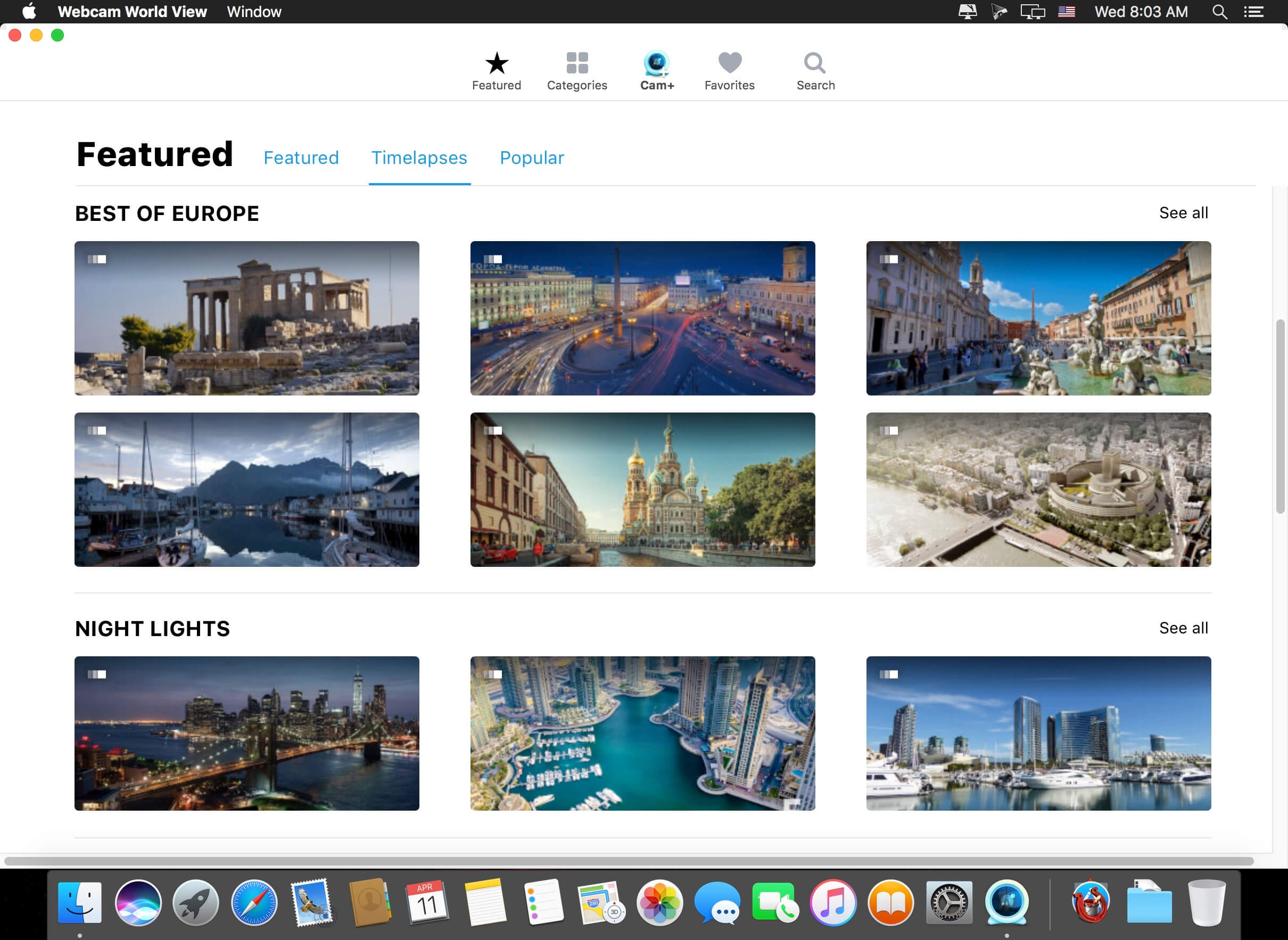Captured on Wednesday at 8:03 a.m., this image showcases an Apple Mac OS X desktop with the Safari browser open. The browser window displays the "Webcam Worldview" webpage. In the upper right-hand corner, there are a few screen notifications, along with a visible search bar and context menu. The webpage features various navigation options including "Featured Categories," "Cam Plus," "Favorite," and "Search" tabs. Below these tabs, there's a menu in black lettering on a white background that highlights options for "Featured," "Time-lapses," and "Popular," with "Time-lapses" being underlined to indicate it is currently selected.

The "Featured" section highlights a "Best of Europe" collection, displaying images from Rome, Sicily, and France. There is also a "Nightlights" section, which features nighttime and daytime views of selected cities. At the bottom of the screen, the taskbar is overcrowded with numerous application icons, making it difficult to distinguish individual applications. This cluttered bar suggests a heavily-used and busy desktop.

Overall, the screenshot effectively encapsulates a typical navigation experience on the "Webcam Worldview" site while hinting at the user's extensive application usage on a macOS system.